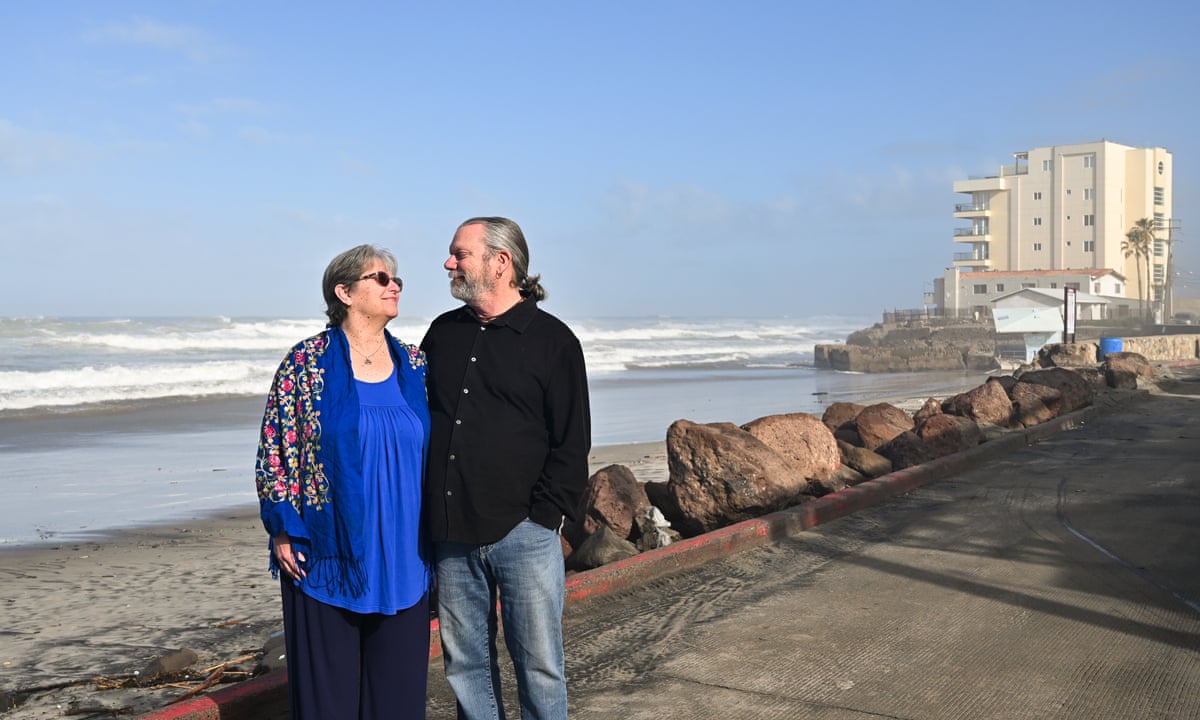In this photograph, two older individuals, likely in their 50s or early 60s, share a tender moment while standing near the beach. On the left, a white woman with short, gray hair is wearing sunglasses, a blue shirt, and a blue silk scarf draped over her shoulders. On the right, possibly her husband, is a man with white hair tied back in a gray ponytail. He is dressed in a black button-down shirt and blue jeans. Both are gazing lovingly at each other.

Behind the couple, the tranquil blue sky forms the backdrop for a picturesque beach scene, where the ocean's waves are visible. To the right, a multi-storied yellow high-rise apartment building, likely a condo complex, stands on a rock ledge with patios that offer sweeping ocean views. A parked car is visible near the building. The couple appears to be standing on a roadway slightly left of center in the composition, enhancing the serene and intimate atmosphere of the scene.